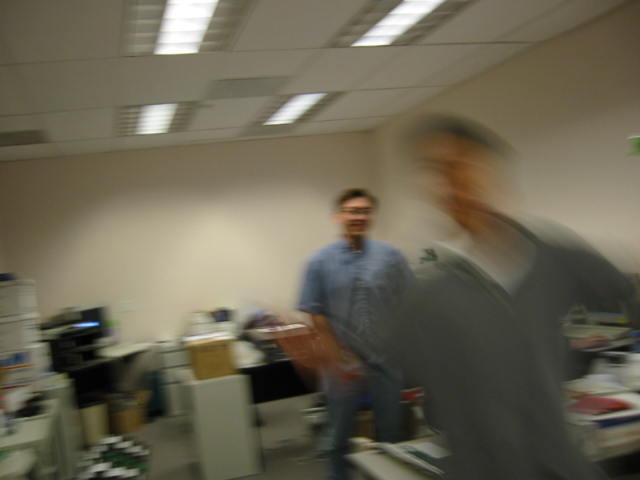In a dimly lit room resembling an office or classroom, the cluttered space features filing cabinets, desks, and stacked boxes scattered around. The ceiling, adorned with white panels, houses square white lights and two gray vents. Beige walls encompass the scene. In the foreground stands a person wearing a gray t-shirt, who appears to be missing their arms. Behind them, another person, dressed in a blue short-sleeved button-up shirt and blue jeans, has black hair and possibly glasses. Among the various items, a black printer with a blue light can be seen accompanied by a couple of brown boxes.